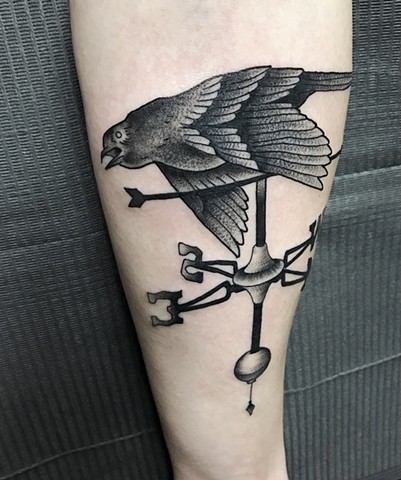This image features a detailed black tattoo set against a gray background, possibly indoors since there's mention of a gray wall or blinds. The tattoo, likely located on the subject's inner arm or thigh, depicts a crow perched atop a weather vane. The weather vane is characterized by its directional markers—north, south, east, and west—indicating it spins in the wind, with an arrow pointing the way. The subject's very pale skin accentuates the dark tattoo, making it the focal point of the image.